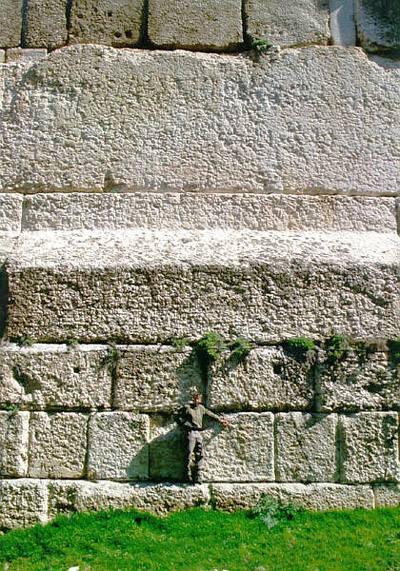This photograph features a man standing against a very tall concrete wall. The wall's base comprises large, stacked concrete blocks, from which green weeds sprout between the seams. A vibrant green grass covers the foreground. Positioned in the center, the man faces the camera, his right arm resting on his hip while his left arm extends to touch the wall. He is dressed in light gray-colored shirt and pants. Above the foundational blocks, a massive rectangular concrete block is prominently visible. Another similar block is positioned above it, showing signs of wear with chipping along the edges. Higher up, the bottom portions of additional concrete blocks, possibly squares, are visible, separated by black seams.